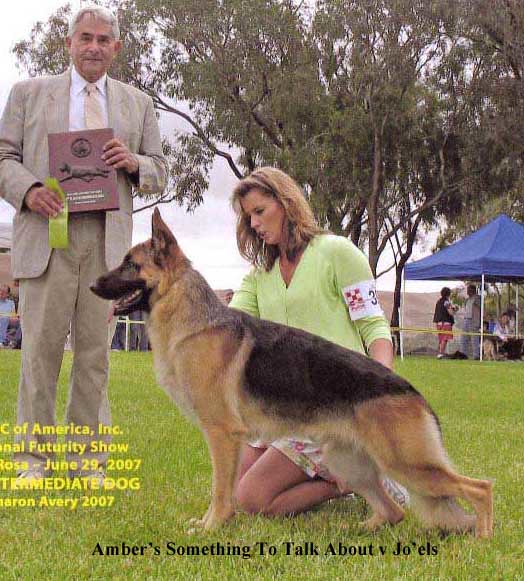The photograph captures a dynamic moment at an intermediate dog show competition in 2007, featuring a poised German Shepherd posed with its hind legs extended and ears alert. The central focus is a woman kneeling on the grass, wearing a light green sweater and an armband with a number, tending and speaking to the German Shepherd. The scene includes a man in a beige suit with white hair and a matching beige tie standing to the left, holding a plaque adorned with a green ribbon, perhaps signifying an award. In the backdrop, a blue tent shelters several onlookers, and beyond a yellow taped line, other spectators and trees can be seen. The woman's name appears to be Sharon Avery. The black text at the bottom reads, "Amber's Something to Talk About v. Joelle's."